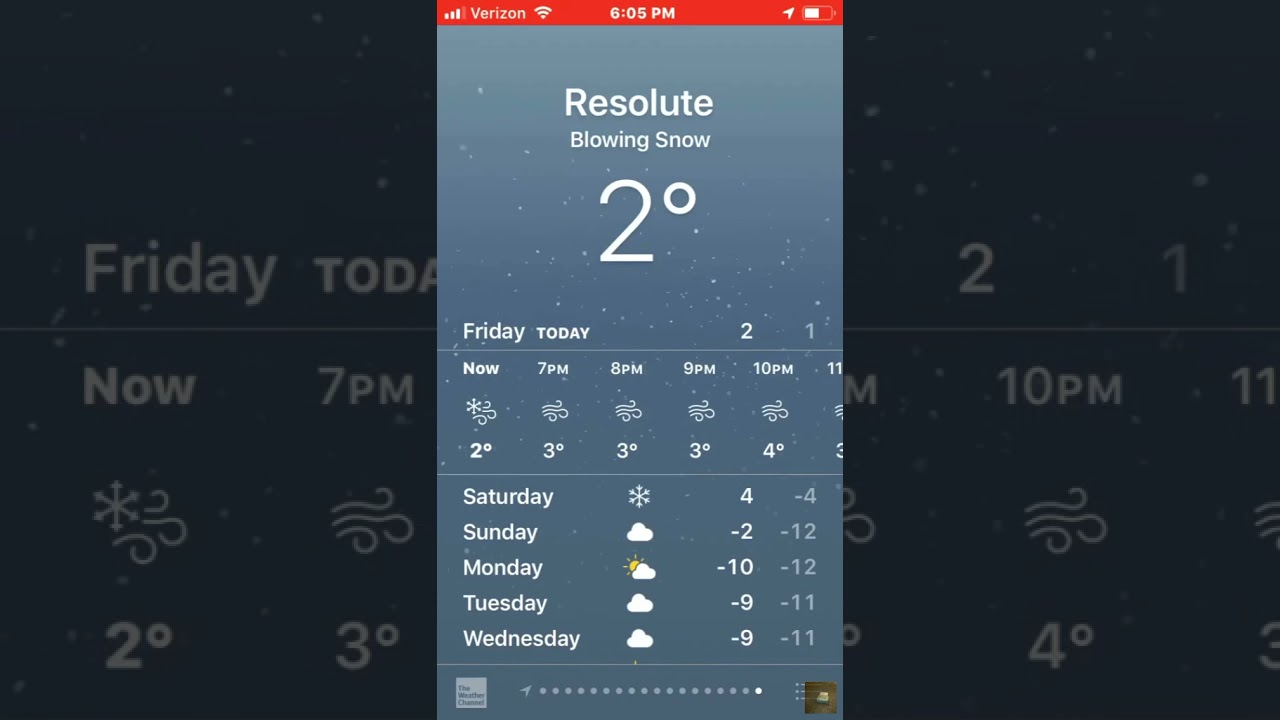The image displays a weather application on a cellphone, indicated by a status bar at the top showing a Wi-Fi signal, the time, battery meter, and the Verizon carrier name. The main interface features a grey background with a heading that reads "Resolute Blowing Snow, 2 degrees". The current weather details are specified below: "Friday", "Today", alongside "Now, 2 degrees" and hourly forecasts: "7pm, 3 degrees", "8pm, 3 degrees", "9pm, 3 degrees", and "10pm, 4 degrees". Underneath, there's an extended weather forecast for the week, listing temperatures: "Saturday, 4 degrees", "Sunday, -2 degrees", "Monday, -10 degrees", "Tuesday, -9 degrees", and "Wednesday, -9 degrees". The entire screen is superimposed onto a larger, slightly blurred image of the same interface, serving as the background wallpaper, creating a layered visual effect.